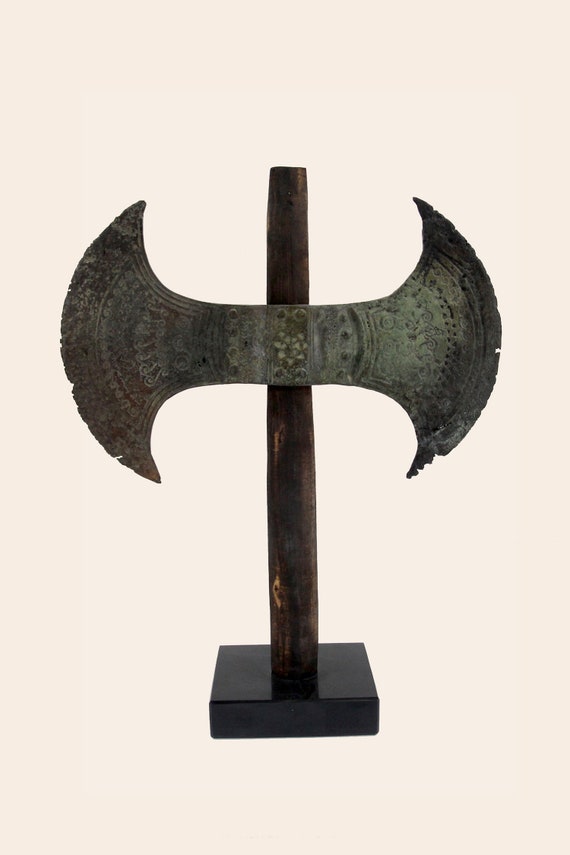The image displays an antique double-headed axe, centered against a pale pink, nearly white background. The axe, made of dark gray metal—possibly black metal or bronze—features sharp, curving blades on either end, which are slightly worn from use. Intricate design patterns radiate from the center outwards. The axe is mounted in an upright position on a black rectangular base, which has a hole for the wooden staff that supports the axe. The staff is simple and straightforward, showing signs of age and use, adding to the weapon's ancient and collectible nature.